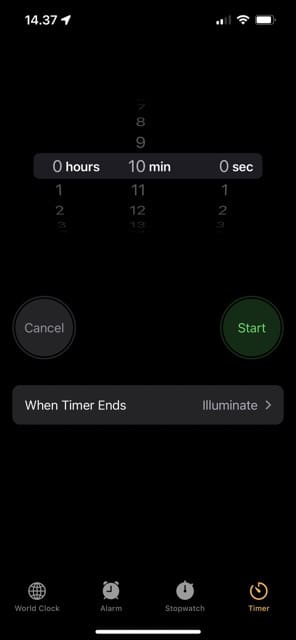The image is a screenshot captured from a mobile device, illustrating the interface of a clock application. At the top of the screen, standard mobile device indicators are visible, including the time, network connection status, Wi-Fi signal strength, and battery level. 

Displayed prominently in the application are four selectable options located along the bottom of the screen: World Clock, represented by a globe icon; Alarm, indicated by an alarm clock icon; Stopwatch, shown with a clock face icon; and Timer, which is currently selected and highlighted in yellow. 

The screenshot reveals the user setting a timer for 10 minutes, with no specified hours or seconds (0 hours, 10 minutes, 0 seconds). Below the timer settings, there are two buttons: a 'Cancel' button and a 'Start' button, the latter of which has a green hue, ready to initiate the timer. An additional note beneath these buttons indicates the timer's action upon completion with the phrase "When timer ends: Illuminate."